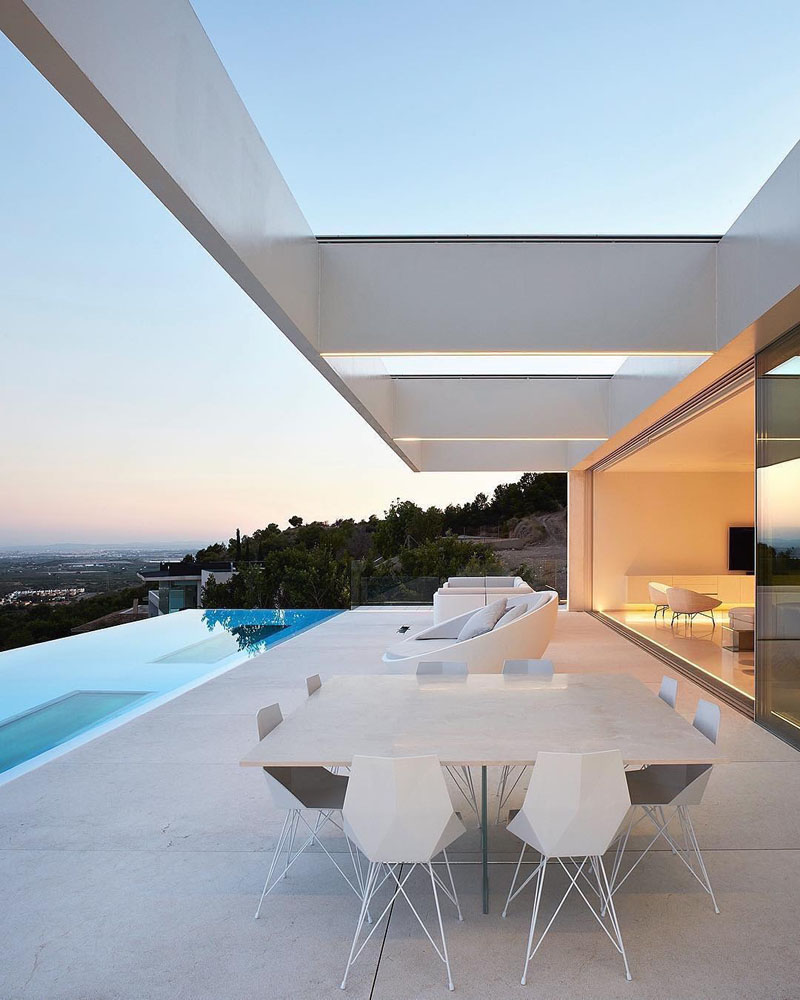The photograph captures the exterior of a modern, luxurious building perched on the side of a mountain. The focal point is a rectangular blue infinity pool that extends outward, offering an unobstructed view of the horizon where the sky transitions from a serene blue to a pinkish hue. Adjacent to the pool is a spacious balcony styled for inside-outside living, featuring a square table surrounded by white chairs. Additional white outdoor furniture, including a chair and a sofa, complements the setting, along with white cushions for comfort. A prominent white beam arches overhead, enhancing the modern aesthetic.

To the right side of the image, through the glass, the softly lit interior glows with a warm orange light, creating a striking contrast with the blue of the pool. The reflection on the glass mirrors the porch setting perfectly. The balcony and pool overlook an urban landscape, possibly Los Angeles, characterized by its modern architectural style and affluence. The natural surroundings include rocks and trees, reinforcing the impression that the house is embedded within a mountainous terrain. The overall scene epitomizes modern contemporary luxury living with breathtaking views.